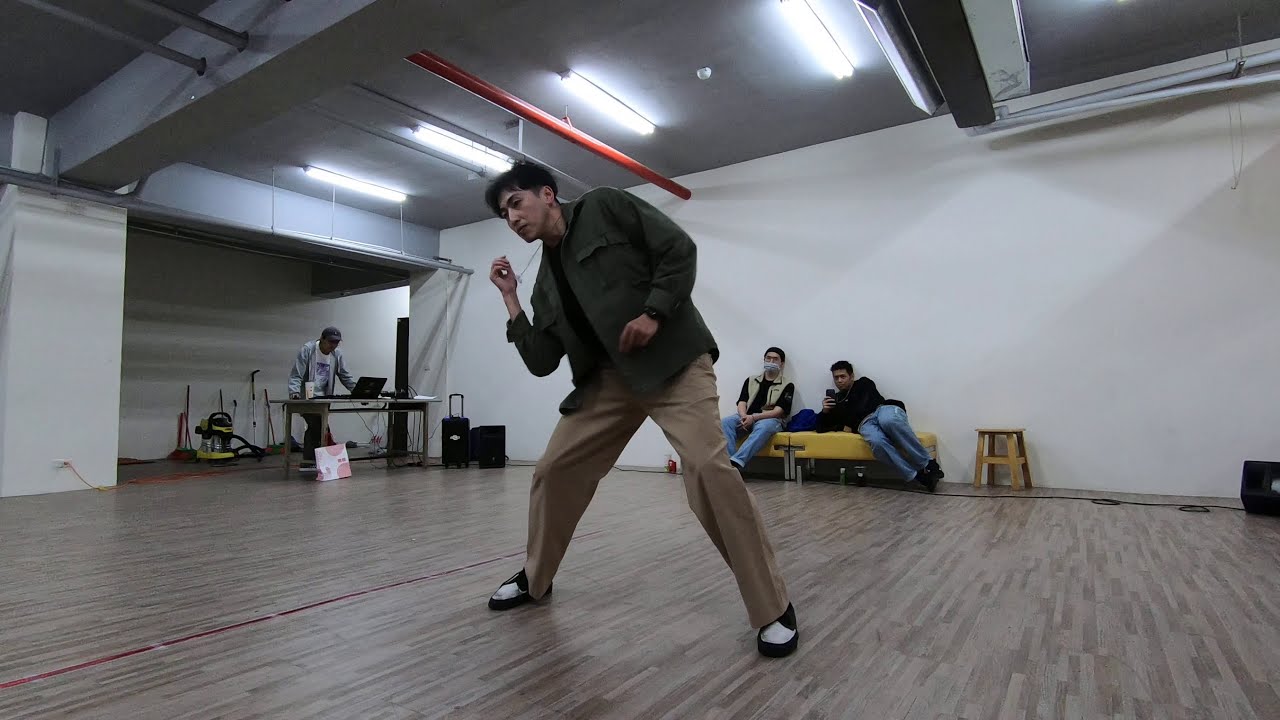In a spacious dance studio with small brown wood panel flooring, an Asian man with short black hair and dressed in khaki pants, a dark-colored button-up shirt, white and black shoes, and a brown coat, is captured mid-dance, moving to the left with one arm raised and leaning sideways. The back wall is painted white with a distinctive red pipe running through the gray ceiling and passing through a gray cement support beam at the center. On this wall, a short yellow bench seats two people, one of whom is wearing a face mask and filming the dancer with a smartphone. Nearby, a low wooden stool sits to the dancer's right. In the background, to the left, a person, possibly a DJ, stands behind a laptop at a desk, surrounded by rolling suitcases. The studio's ceiling features large metal air-conditioning ducts and four bright fluorescent lights, illuminating the room uniformly. Additionally, a red wire is visible on the floor, taped down with white tape, running straight through the center of the room.